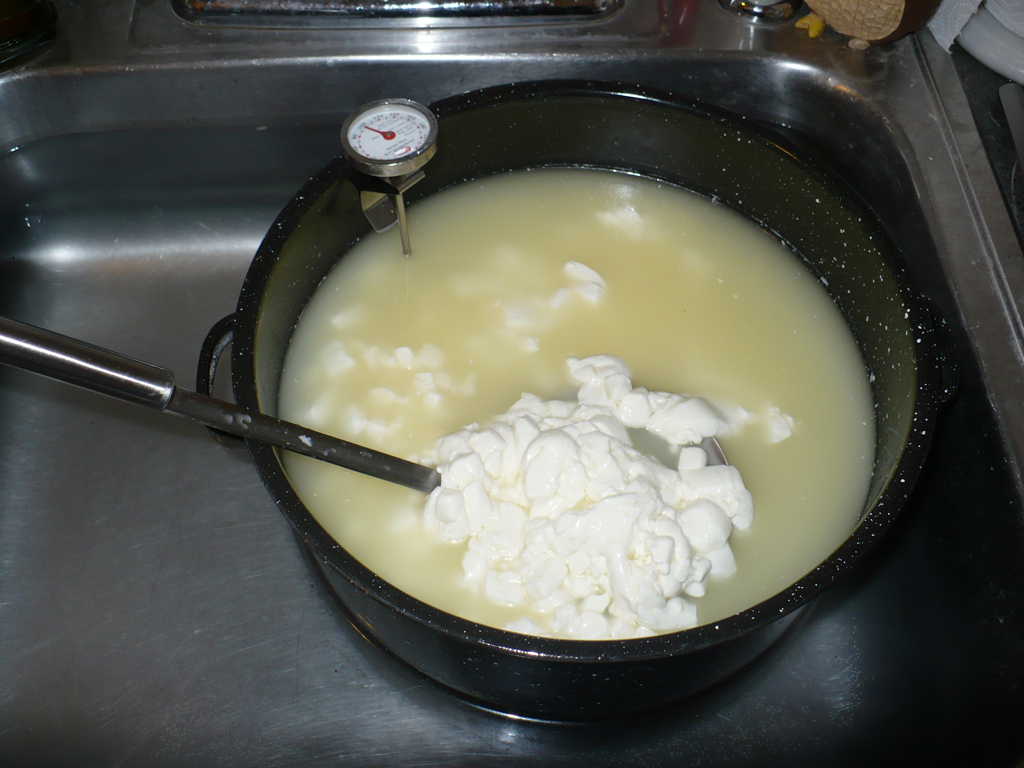The image showcases a detailed scene of a culinary process taking place in a dimly lit kitchen. At the center of the photograph is a substantial black pot adorned with small white speckles, equipped with small handles on either side. The pot is carefully placed inside a stainless steel sink that is partially filled with water. Inside the pot, a thin, yellowish-brown liquid surrounds substantial chunks of a thick, white, curdled substance, resembling cottage cheese or ricotta.

A long silver ladle, resting on the pot's edge, is used to scoop up the chunky material, lifting it above the liquid's surface. Additionally, a metal thermometer is clipped to the pot's rim, its probe dipping into the broth to monitor the temperature. Various kitchen items such as knick-knacks and a roll of paper towels can be seen in the background, adding to the amateur, home-cooking vibe of the photograph. The collective elements suggest that the process depicted might be related to cheese-making or similar culinary preparation.